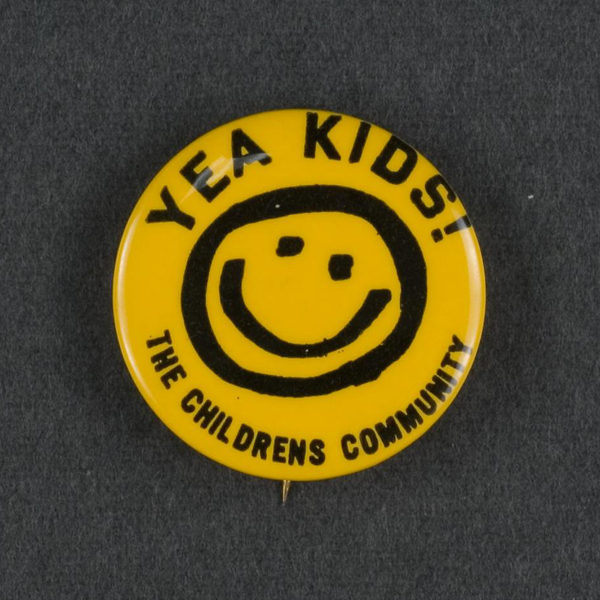The image features a circular yellow button designed to be affixed to clothing, positioned upright on a soft, padded, gray fabric background. The button prominently displays a cheerful yet asymmetrical smiley face illustration in the center. Above the smiley face, in playful, black print lettering arranged in a semi-circle, are the words "Yay kids!" At the bottom, also in black lettering forming a semi-circle, it reads "The Children's Community." The button has a simple, childlike design with a slight sheen from a plastic cover, and a glimpse of the pin mechanism is visible at the bottom. The button is the sole object in the image, and the overall setup suggests it could be part of a product listing or personal item depiction.